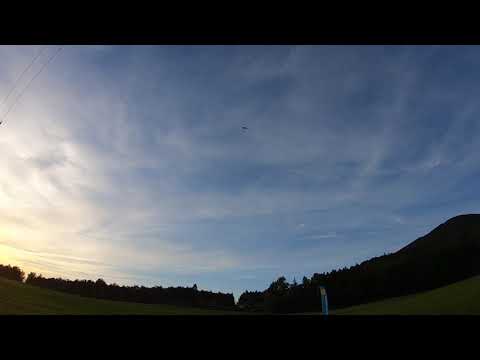This horizontally aligned, rectangular photograph showcases a serene outdoor landscape framed by thick black borders at the top and bottom. In the lower part of the image, a verdant expanse of green grass stretches across from left to right, dipping gently to form a subtle valley at the center. The grass edges upward to the left and right, flanked by a dense row of trees with abundant green leaves, appearing almost as a continuous silhouette due to the subdued lighting.

Above this lush foreground, the expansive sky dominates the scene, characterized by a harmonious blend of blue hues interspersed with light gray and white, feathery clouds. The sky's brightness intensifies toward the upper left, hinting at the hidden sun behind a brighter patch of clouds. In the upper left corner, two power lines subtly intersect the serene atmosphere. At the center of the sky, a tiny bird in flight adds a delicate focal point. Additionally, towards the right of the center, a vaguely discernible blue object, possibly a pole, punctuates the horizon. The overall photograph, although slightly darkened, exudes a tranquil, pastoral beauty with its interplay of light and shadow.